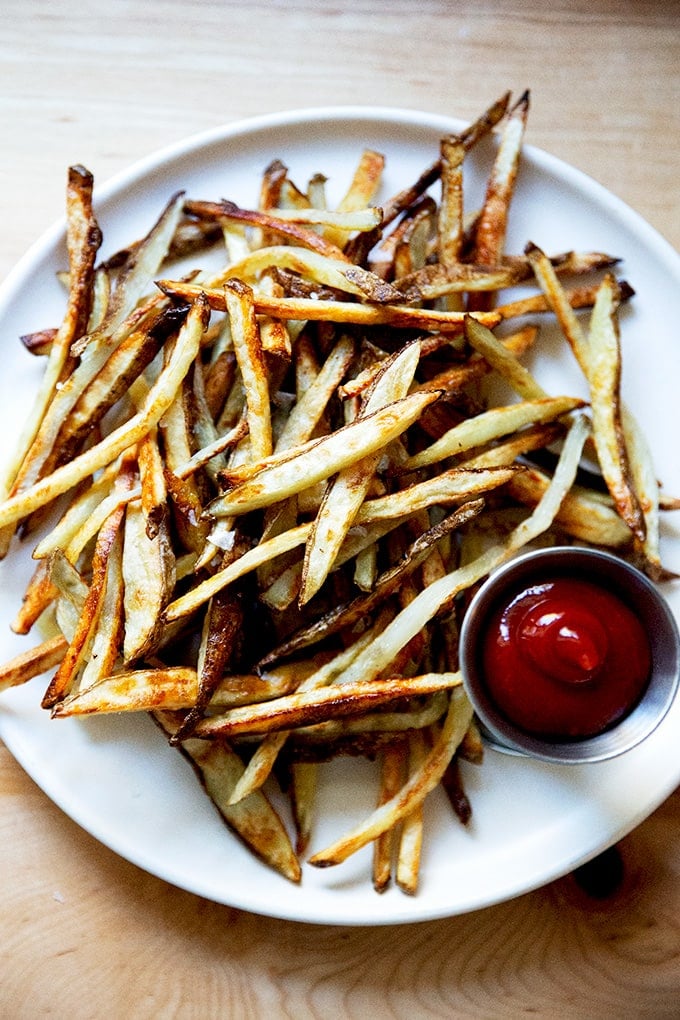An overhead food portrait captures a tempting pile of homemade, shoestring-sized french fries heaped onto a simple white plate, set atop a light-colored wooden table. The fries, irregular in size and color, display a range of hues from golden yellow to crispy dark brown with visible potato skin on some. Their edges are golden brown, while others exhibit a more burnt and crispy texture. Prominently featured to the front right of the plate is a round silver serving dish filled with ketchup, topped with a perfectly peaked swirl. The table's wood grain texture can be seen clearly at the bottom right of the photo, and sunlight from the top illuminates the scene, enhancing the inviting look of the fries.